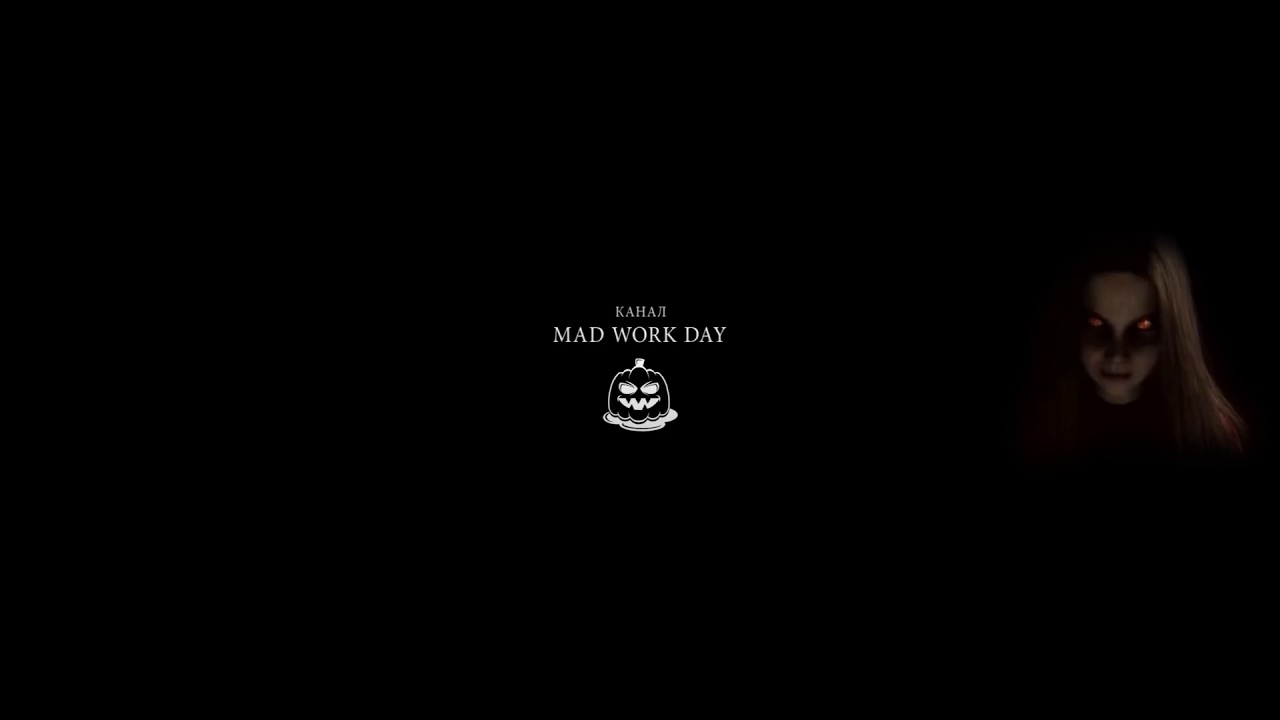The image is a photographic-style poster with a predominantly black background, set indoors. Centrally positioned text in white reads "K-A-H-A-J-I" followed by "Mad Workday" in a slightly larger font. Below this text, there's a graphic of a jack-o'-lantern on a platter, displaying a sinister smile. To the right side of the image, there is a detailed portrayal of a young white woman with long hair cascading past her shoulders. Her face is slightly elongated with a prominent chin and covered in black sunglasses. Her expression is unsettling, with details suggesting she could appear possessed or malevolent, including dark circles around her eyes and a downward gaze. The overall composition is eerie and mysterious, reminiscent of a horror movie poster or an advertisement, highlighted by the stark, ominous atmosphere and minimal yet striking visual elements.